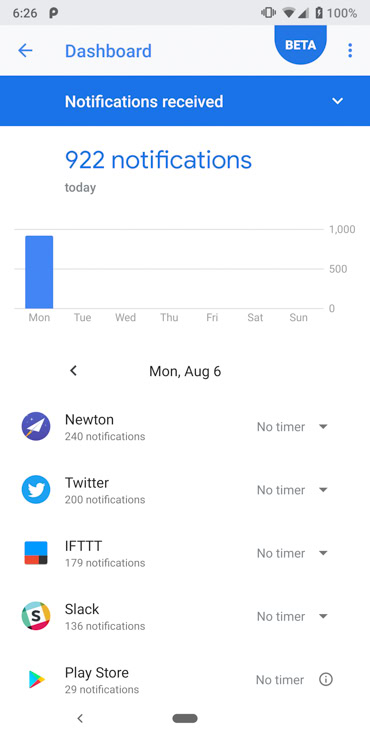The image is a screenshot of a smartphone screen taken at 6:26 PM. In the upper-left corner, the time "6:26 PM" is displayed. On the opposite side, icons for Wi-Fi reception and a fully charged battery (100%) are visible. Below these icons, there is a blue text reading "Dashboard" accompanied by a left-pointing arrow, and adjacent to it is the word "Beta" followed by three vertical dots.

A prominent blue banner or button below this text reads "Notifications Received" with a downward arrow beside it. Against a white background, it is noted that there are "922 notifications today." 

A chart is also visible, mapping the number of notifications received each day of the week, with a vertical axis on the right indicating the number of notifications. 

Below the chart, specific data for Monday, August 6, is listed, showing notifications received from various sources: Newton received 240 notifications, Twitter received 200 notifications, IFTTT received 179 notifications, Slack received 136 notifications, and the Play Store received 29 notifications.